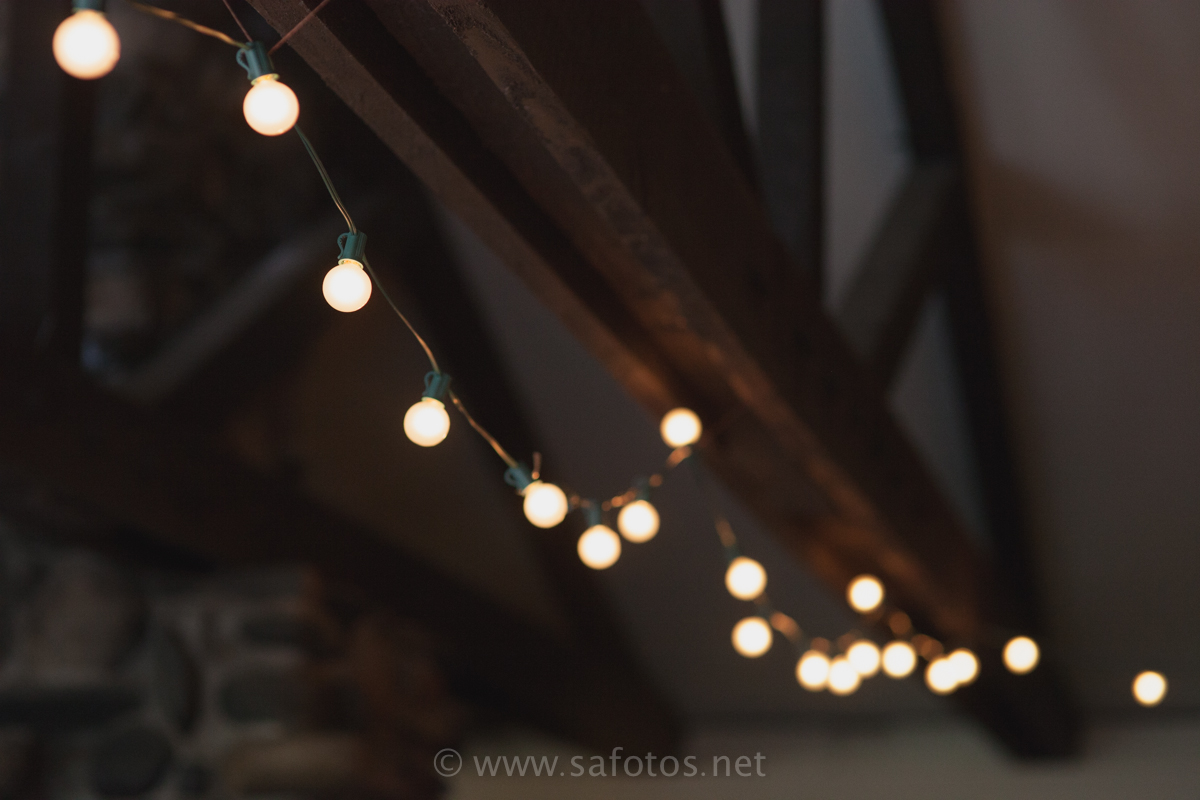This image captures an outdoor setting, likely a deck area, adorned with numerous small, circular lights that bear a resemblance to tiny grapes or Christmas lights. These lights are strung together, creating a delicate, festive atmosphere. Mounted onto a wooden structure, the lights emit a warm, inviting glow that enhances the serene ambiance of the outdoor space. At the bottom of the image, there is text that features a website, www.safotos.net, along with copyright information.